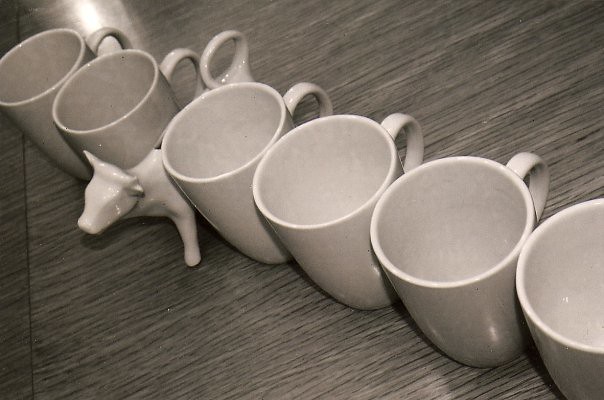The image features a neat row of six white ceramic coffee mugs, all identical in their simple design, placed closely together on a dark gray wooden surface. The uniformity of the mugs is broken by an unusual addition between the fourth and fifth mugs: a white ceramic piece resembling a bull or ram. This ceramic figure has a tail that curves like a handle, suggesting it might be functional, possibly used for pouring or even as a whimsical drinking vessel. The gray surface could be a table, countertop, or floor, adding a neutral backdrop that complements the mugs and the unique ceramic animal.